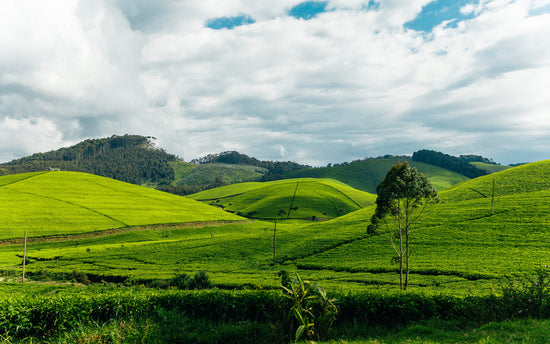The photograph captures a picturesque scene of terraced plantations on rolling, dome-like mountains, reminiscent of Indian burial mounds, with meticulously divided green sections creating an almost artistic pattern on the hills. The foreground hills are sparsely wooded, showcasing well-groomed grass, while the more distant mountains on the horizon are dotted with various trees and dense forests, adding depth to the landscape. The tranquil ambiance is enhanced by the partly cloudy sky, with sunlight softly illuminating the verdant fields, making the entire setting appear peaceful and serene.